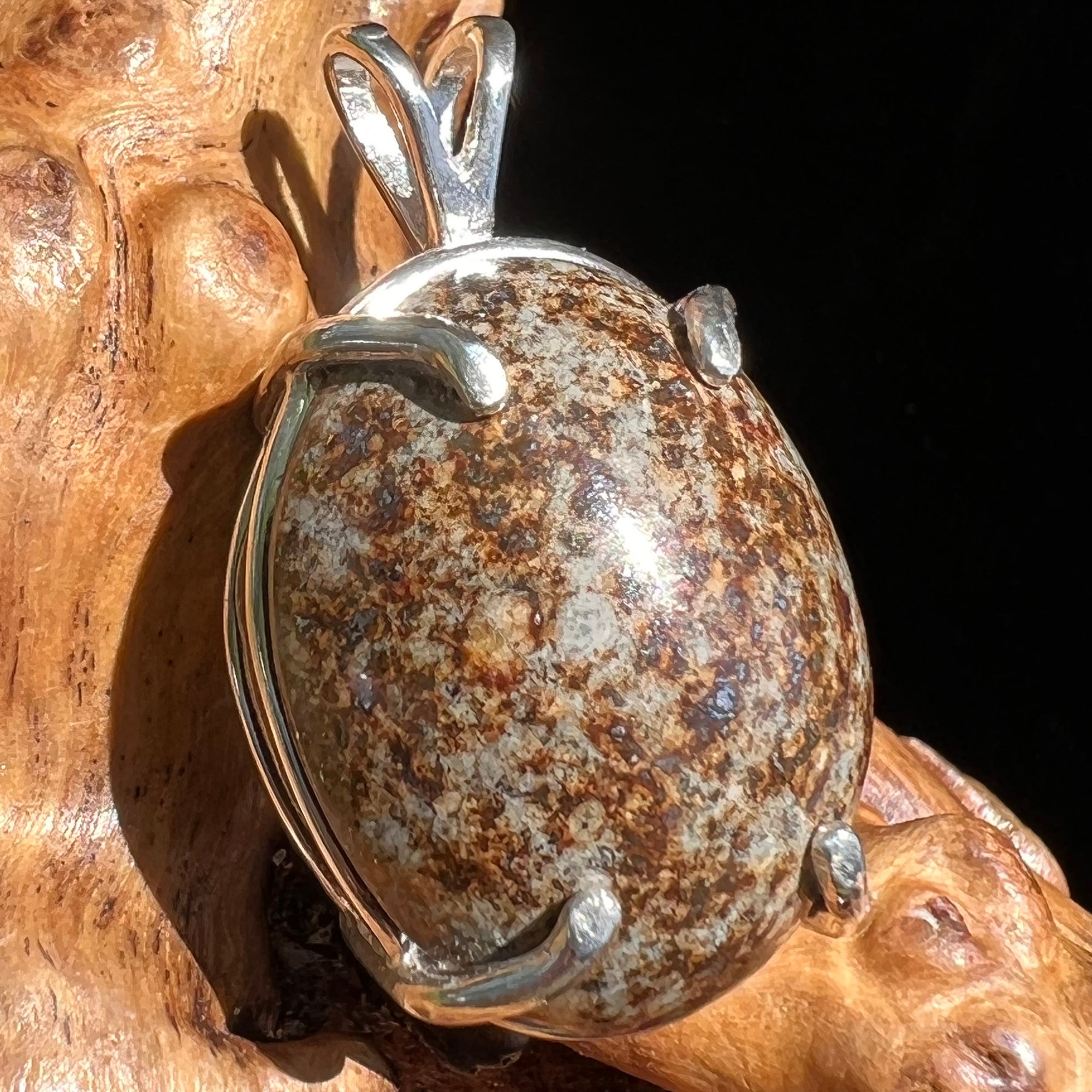This detailed close-up photograph captures an intricately designed piece of jewelry, likely meant for a necklace, lying on a smooth, polished wooden surface. The centerpiece of the image is an oval-shaped, polished stone with a speckled appearance, featuring hues of gray, brown, tan, beige, and a hint of green. The stone’s texture almost resembles an alien planetary terrain, adding to its exotic charm. It is securely held in place by a silver clasp with four prongs—two at the top and two at the bottom—giving it an arm-like look. At the top of the clasp, there is a double eyelet or bow, designed to fit a silver chain, although no chain is present. The surrounding background is a deep, uninterrupted black, creating a striking contrast that draws attention to the natural beauty of the stone and the craftsmanship of the silver setting. The wooden surface underneath, possibly a tree that has been trimmed, sanded, and varnished, exhibits smooth, bread-like textures with darker brown lines and subtle white reflections, adding another layer of natural elegance to the composition.